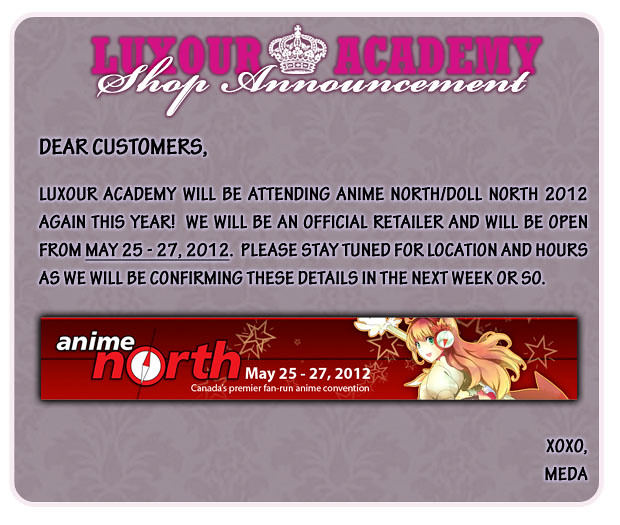The image is a square with a rounded top and a patterned background in a grayish-brown color, featuring a paisley design. At the top, in dark pink letters, it reads "Luxor Academy" with a white crown outline between the two words. Below that, in white cursive, it says "Shop Announcement." Left-aligned and in black capital letters, it reads "Dear Customers." The text underneath announces that "Luxor Academy will be attending Anime North/Doll North 2012 again this year. We will be an official retailer and will be open from May 25th to 27th, 2012. Please stay tuned for location and hours as we will be confirming these details in the next week or so. XOXO, Meta Hamikiya." 

A horizontal rectangular section in dark red with black lines features additional event details. In the upper left corner, in white letters, it says "Anime North." Below that, "North" is spelled out with a white 'O' and red letters for the rest. Centered, it lists the dates "May 25th-27th, 2012." On the right-hand side, there's an image of an anime woman with long pink and blonde hair, surrounded by stars. This section also includes a note stating that Anime North is Canada's premier fan-run anime convention.